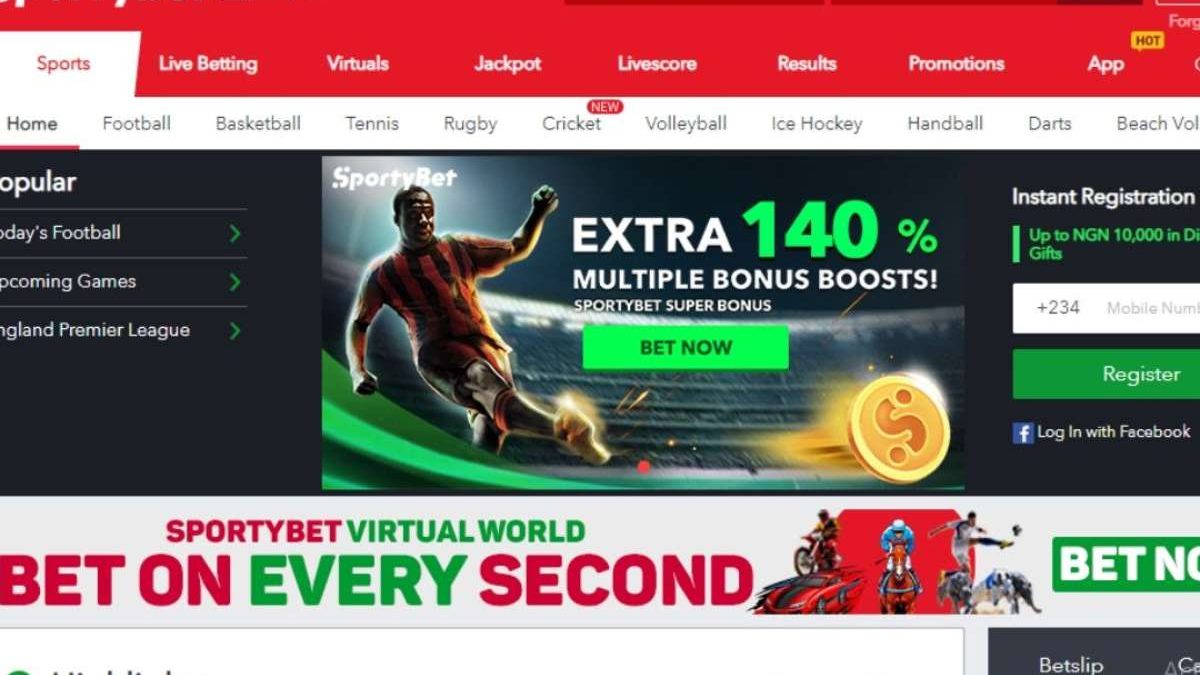The web page features a prominent red rectangle at the top with white text labels including "Live Betting," "Virtual," "Jackpot," "Live Scores," "Results," "Promotions," and "App." A small yellow "Hot" speech bubble design adds a highlight to the top section. Immediately below, a larger white rectangle with the word "Sports" in red precedes a black-on-white menu listing: "Home," "Football," "Basketball," "Tennis," "Rugby," "Cricket," "Volleyball," "Ice Hockey," "Handball," "Darts," and "Beach Ball." The left side cuts off some text revealing partial words like "opular" for "Popular," "days football" for "Today's Football," "P coming games" for "Upcoming Games," and "NGLAND premier league" for "England Premier League."

An illustration of a person appears to be kicking a ball, accompanied by promotional text stating "Extra 140% Multiple Bonus Boost," "Sports Bet Super Bonus," and "Bet Now." Options for "Instant Registration" and login via Facebook are also displayed. Users can enter their mobile numbers and encounter an additional ad touting "Sporty Bet Virtual World – Bet on Every Second," featuring images of people on bicycles, kicking a ball, and possibly huddling. The phrase "Bet Slip" is placed over a black-and-white color scheme at the bottom.